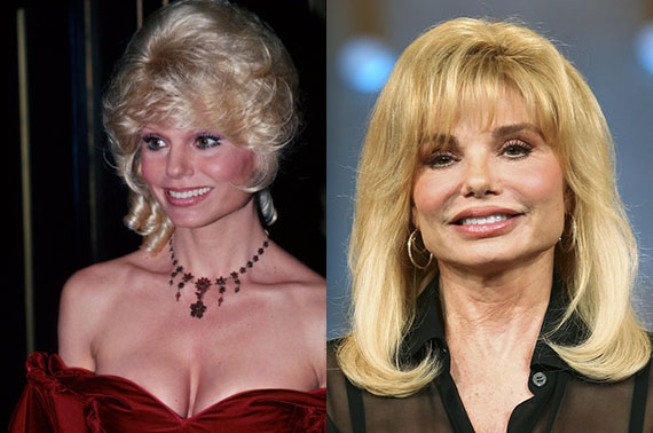The image features two side-by-side, professionally taken photos of the well-known actress Lonnie Anderson at different points in time. In the left photo, a younger Anderson is depicted with yellowish blonde hair styled glamorously. She is adorned in a low-cut, off-the-shoulder dark red satin or velvet dress, accessorized with a striking beaded necklace featuring red and black gems and flowered patterns. The background behind her is dark with indistinct lines. On the right, a more current image of Anderson shows her with her hair down and shoulder-length, wearing thin gold hoop earrings. She is dressed in a sheer black button-down blouse that is open at the collar, smiling and looking at someone off-camera. The backdrop in this image is a blurred variety of blue shades. Both images exude a sense of elegance and capture her timeless beauty.